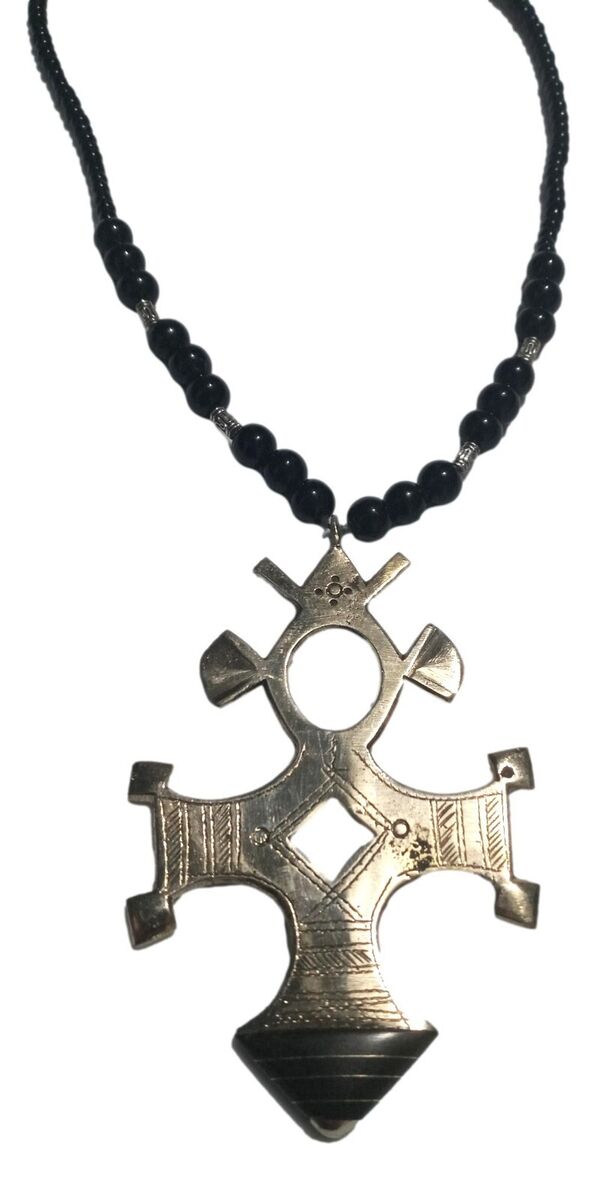The image features a detailed photograph of a handcrafted African Tuareg Berber cross necklace set against a featureless white background. The necklace is predominantly black, with both the cord and the beads sharing this color. The beads are arranged in groups of three on either side of the pendant, totaling eighteen beads. The pendant itself is an intricate, highly elaborated cross-like shape, exhibiting a blend of geometric and ornamental designs. The top arm of the pendant is diamond-shaped with a circular hole in its center, while the bottom arm features a solid black section adorned with stripes and inlays. The pendant's sides are decorated with triangular and metal square extrusions, creating a unique, slightly bent appearance. The overall craftsmanship of the pendant suggests a handcrafted quality, giving it a distinctive, culturally rich aesthetic. The photograph is black and white, emphasizing the detailed artistry and heaviness of the necklace.